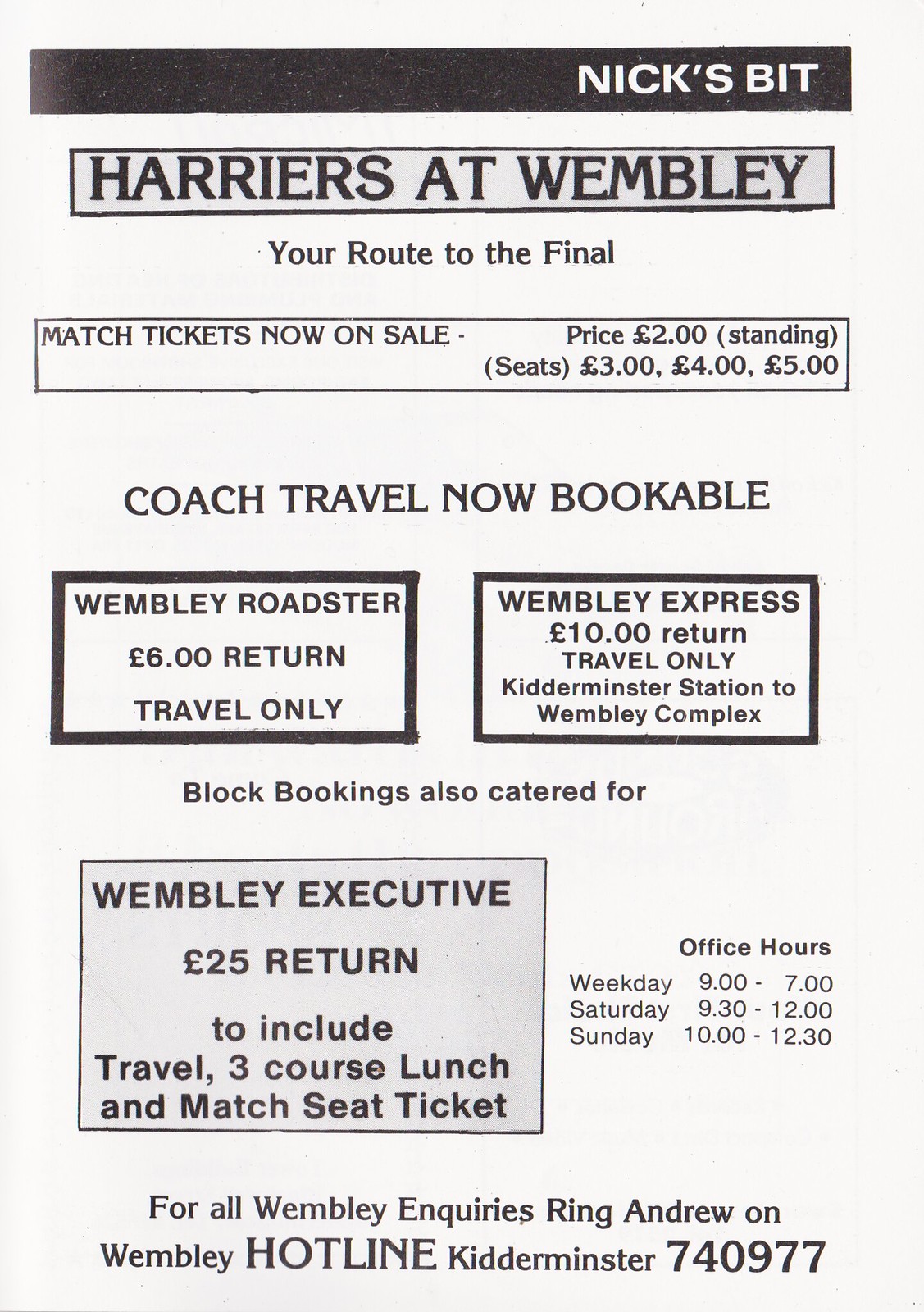The image is a detailed advertisement pamphlet titled "Nick's Bit" prominently featured at the top with a black bar and white text on the right side. Below it, a square highlights "Harriers at Wembley" in black text with a black outline, followed by the tagline "Your final route to the final." Listed beneath are match ticket prices: standing tickets at $2.00, seats priced at $3.00, $4.00, and £5.00. It also mentions coach travel availability.

There are two adjacent squares detailing travel options: "Wembley Roadster" at £6.00 return (travel only) and "Wembley Express" at $10.00 return (travel only), from Kidderminster Station to Wembley Complex. Another square with a grey background promotes "Wembley Executive" at $25.00/£25.00 return, which includes travel, a three-course lunch, and a match seat ticket. Office hours are specified as Wednesday 9-7, Saturday 9:30-12, and Sunday 10-12:30. For Wembley inquiries, it directs to call Andrew on the Wembley Hotline at Kidderminster 740977. The overall design features a white background with black text, and some sections boxed with black shading.